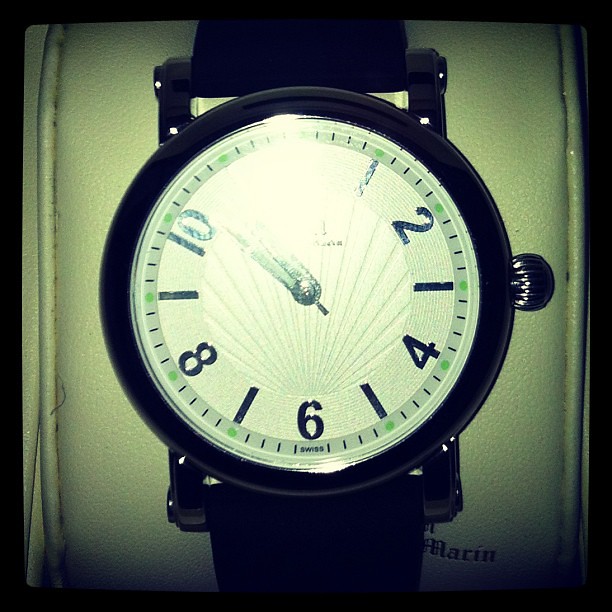The image showcases a wristwatch positioned on a white leather background, clearly displaying the brand name "Marin" stitched in black on the leather. The watch features a sophisticated design with a reflective black or silver metal case and a prominent white face, which bears black numerals and minute markings. Notably, the watch displays numbers at the 1, 2, 4, 6, 8, and 10 o'clock positions, while the 3, 5, 7, 9, and 11 are represented by black dashes with small green dots at the outer edge. The timepiece has a visually striking center design resembling a scallop shell, radiating lines outward from above the 6 o’clock position. Unfortunately, a bright camera flash obscures the 11 and 12 o’clock positions, as well as the hands of the watch, which appear slightly past the 10 o'clock mark. The watch is encircled by a black trim with a functional winding knob on the right side, and it is affixed with a matching black strap.